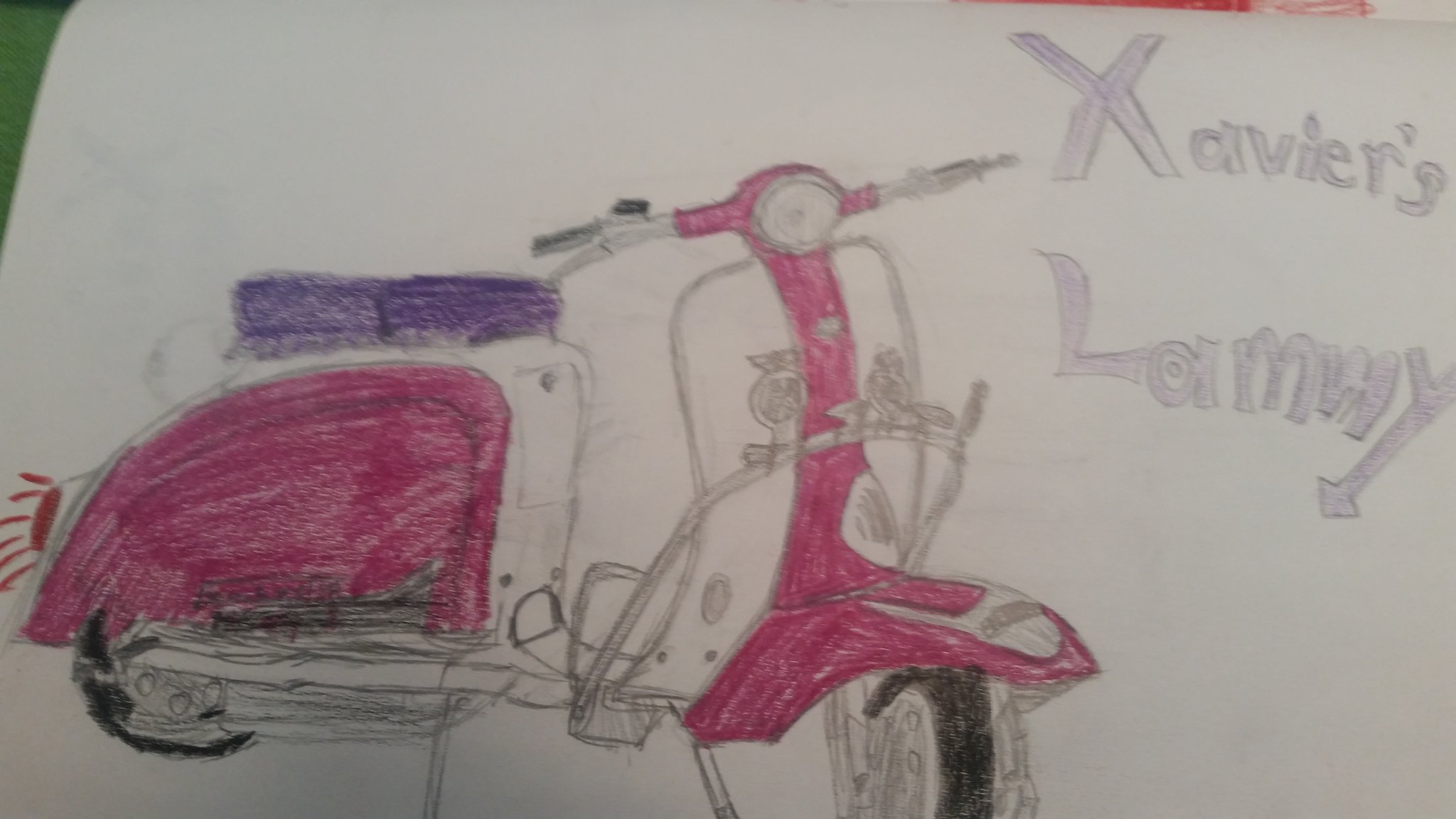This artwork depicts a meticulously drawn moped, reminiscent of a classic Vespa, on stock white paper. The primary focus is on the moped, which features vibrant pink coloration with a contrasting purple seat, all rendered using colored pencils. The scene is minimally detailed, allowing the viewer to appreciate the intricacies of the moped itself. Notably, the taillight glows subtly, indicated by small light dashes. The moped rests on a sturdy kickstand, suggesting it is stationary. In the background, faint traces of another image peek through, with hints of white and red, although they are unrelated to the main subject. To the right of the drawing, the text "Xavier's Lammy" identifies the moped. The tires are shaded in black, adding a touch of realism, while the rest of the drawing remains uncolored, emphasizing the detailed, classic moped design.